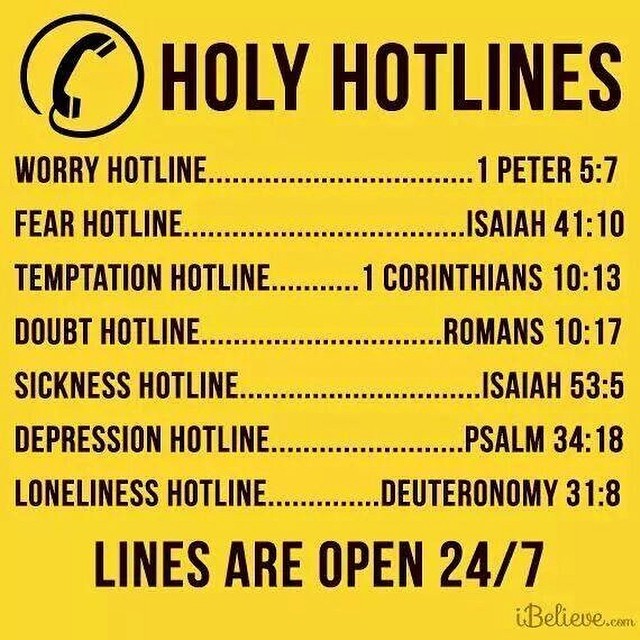The image features a yellow background with black text and is digitally created. At the top, there is a black telephone icon inside a circle. Right next to it in the largest, dark brown font, it reads "Holy Hotlines." The center of the image lists various hotlines, each aligned left and right with dots connecting them to their biblical references. The hotlines include:

- **Worry Hotline:** 1 Peter 5:7
- **Fear Hotline:** Isaiah 41:10
- **Temptation Hotline:** 1 Corinthians 10:13
- **Doubt Hotline:** Romans 10:17
- **Sickness Hotline:** Isaiah 53:5
- **Depression Hotline:** Psalm 34:18
- **Loneliness Hotline:** Deuteronomy 31:8

At the bottom of the image, large black text declares "Lines are open 24-7." In the lower right corner, in a lighter black cursive font, it reads "Ibelieve.com."